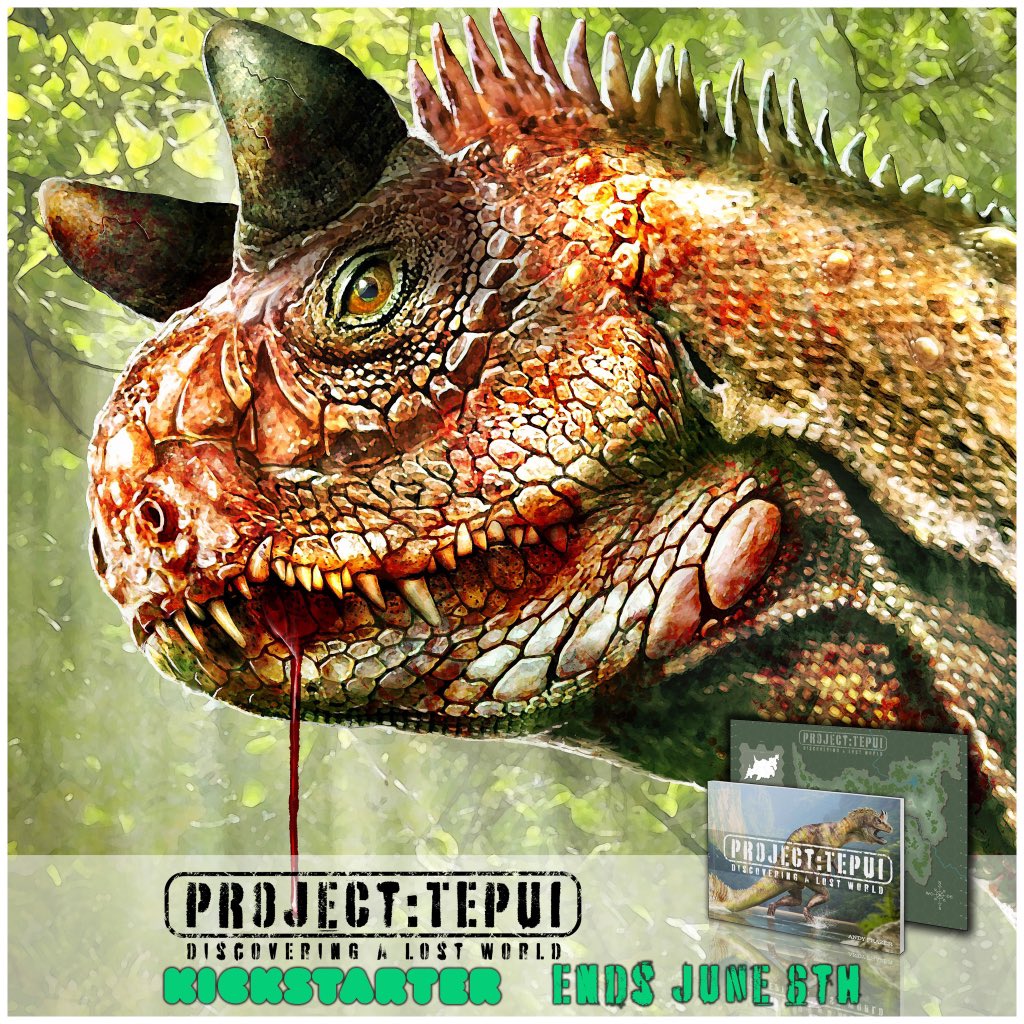The header image for the Kickstarter campaign "Project Tepui: Discovering a Lost World" is vibrant and eye-catching. Central to the image is a watercolor painting of a prehistoric reptile, an unfamiliar species resembling a blend between an iguana and a dinosaur, with black horns adorning the top of its head. The creature's face exhibits striking colors—reds, oranges, and yellows—complemented by piercing red eyes. Blood drips menacingly from its visible canine teeth, enhancing its fierce appearance. The backdrop is a lush green forest, creating a sense of deep jungle mystery. The bottom of the image features the campaign's title and the end date, June 6, in a mix of bold green and weathered black fonts. Additionally, smaller thumbnails in the image display a product box and a world map, both branded with "Project Tepui: Discovering a Lost World." A subtle inclusion in the corner shows a Tyrannosaurus rex, tying the project further to its prehistoric theme.